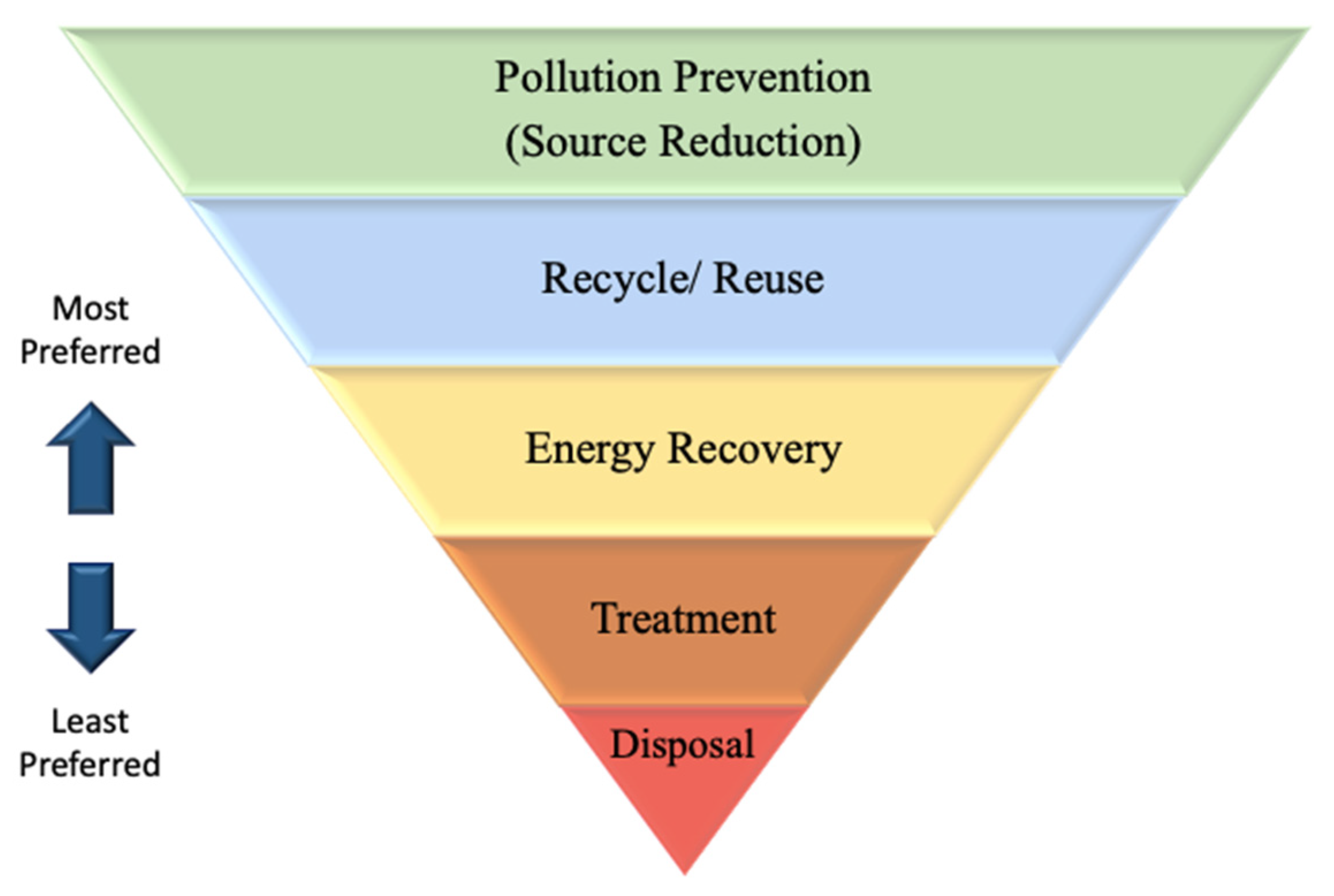The image is a simple computer-generated infographic with a white background, showcasing an inverted pyramid that illustrates the hierarchy of waste management practices aimed at reducing pollution and caring for the environment. The pyramid is divided into five color-coded layers, each representing a different strategy, starting from the most preferred at the broad top to the least preferred at the narrow bottom. The top green layer is labeled "Pollution Prevention (Source Reduction)," followed by a blue layer labeled "Recycle/Reuse," a yellow layer titled "Energy Recovery," an orange layer marked "Treatment," and finally, at the very bottom, a red layer labeled "Disposal." All text is in black serif font. On the left side of the pyramid, two arrows indicate the preference hierarchy, with "Most Preferred" at the top and "Least Preferred" at the bottom. Blue arrows reinforce the direction from the top of the pyramid to the bottom, clearly emphasizing the prioritization of waste management methods.